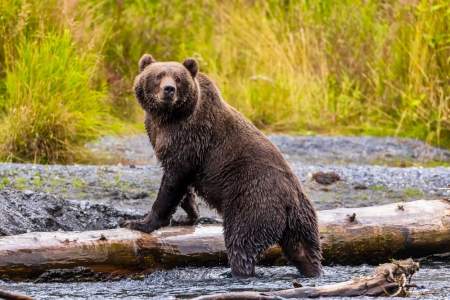In this captivating outdoor scene captured in a color photograph, a large, dark brown bear, commonly referred to as a black bear, is the central focus. The bear rests its front paws on a horizontal log, half-submerged in greyish-brown mud or water, while its rear legs extend behind it. The bear's body is turned away from the camera, but it looks back over its left shoulder, directly at the viewer. Its wet fur, darker around the body and lighter around the muzzle, glistens, adding texture to the scene. The bear's ears, small half-circles, are perked up above its head. Surrounding the bear, the background features lush, green, and yellow foliage in softer focus, enhancing the natural, serene atmosphere. A smaller, submerged branch is also visible near the main log. The overall composition, with the bear's attentive gaze and the vivid greenery, creates a striking image of wildlife in its natural habitat.